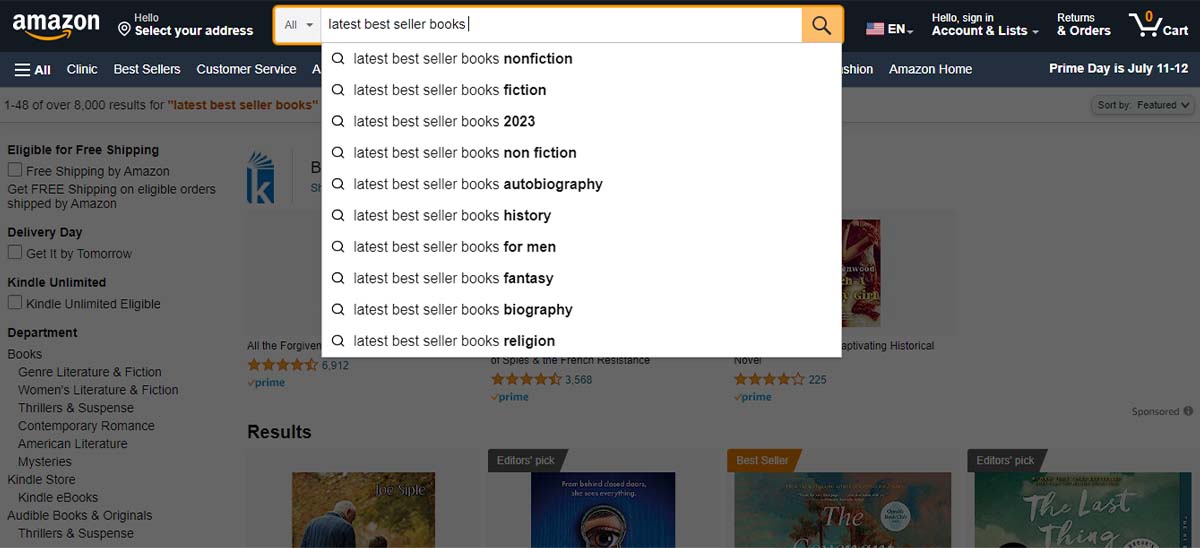This image is a screenshot of an Amazon webpage. At the very top, there's a distinctive black navigation bar extending horizontally across the screen. On the left side of this bar, the recognizable Amazon logo is prominently displayed. Adjacent to the logo, the text reads, "Hello, select your address."

In the central portion of the black bar is a search area. The search bar features a drop-down menu labeled "All" on the left side. The text "Latest Bestseller Books" is typed into the search field, indicating a user's current search query. Beneath the search bar, a drop-down menu is open, displaying approximately ten autofill search suggestions, each beginning with "Latest Bestseller Books." The suggestions include various categories such as Nonfiction, Fiction, 2023, Nonfiction (repeated), Autobiography, History for Men, Fantasy, Biography, and Religion.

To the right of the search bar, additional navigation options are visible. There's a drop-down menu labeled "EN" for language selection, followed by the prompt "Hello, sign in." This is linked to an accounts and lists drop-down menu. Further along, there is a "Returns & Orders" button and a shopping cart icon.

Overall, the screenshot captures a typical Amazon search interface, focusing on books, with several user-specific options and navigational features.